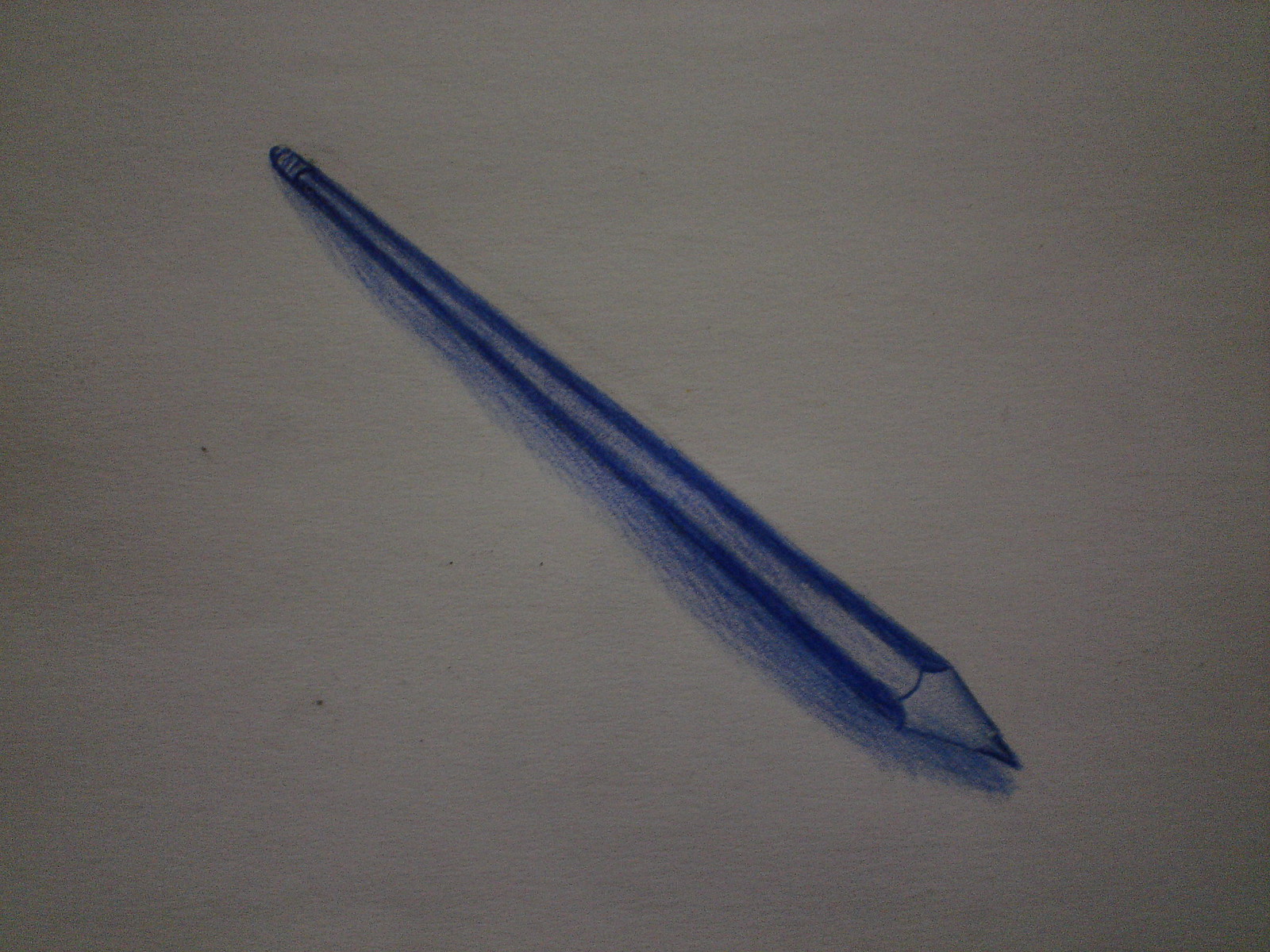A meticulously rendered drawing captures a blue pencil in fine detail. Created with either a blue colored pencil or a skillfully used Bic pen, the artwork showcases a realistic representation with soft shading and intricate line work. The pencil is depicted lying diagonally on a plain sheet of paper, with the eraser end positioned towards the upper left corner of the composition and the sharpened lead pointing towards the bottom right. Noticeable shadows beneath the pencil suggest a light source from above, although the highlights on the pencil itself lack consistency. The overall ambiance of the scene appears quite dark, casting ambiguity on whether the paper itself is tinted or if the photograph of the drawing was taken in low light conditions.